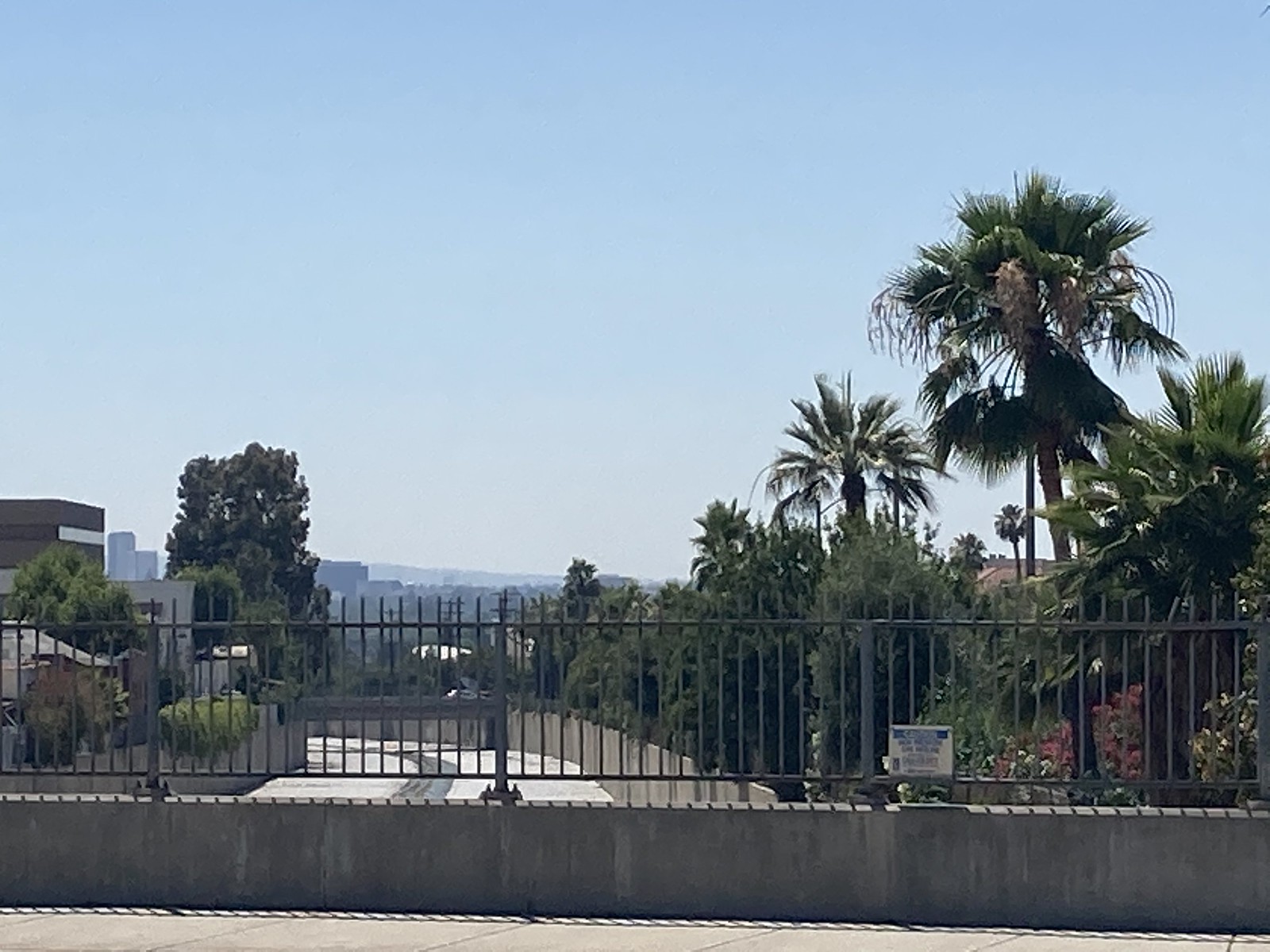The image captures a scenic overlook, likely from an elevated position such as a bridge. Dominating the foreground is a black metal fence, providing a point of reference for the viewer's vantage point. Below, a light grey concrete path or road curves gracefully to the left, winding its way from underneath the bridge. To the right of this road, a row of stately palm trees adds a touch of tropical charm, contrasting with the diverse array of trees that line the left side.

In the midground, a cluster of buildings is visible, varying in size and function. On the left side, these structures include both taller edifices and smaller residential houses, potentially indicating a mix of flats and homes. Beyond these buildings, the urban landscape transitions to include a few high-rise buildings that punctuate the skyline.

The backdrop is crowned with distant mountains or hills, providing a natural boundary to the horizon. The expansive blue sky occupies the top two-thirds of the image, creating a serene and open atmosphere, with the upper reaches of the trees gently interrupting the sea of blue. This detailed composition offers a harmonious blend of natural and urban elements, framed by the elevated perspective of the photographer.